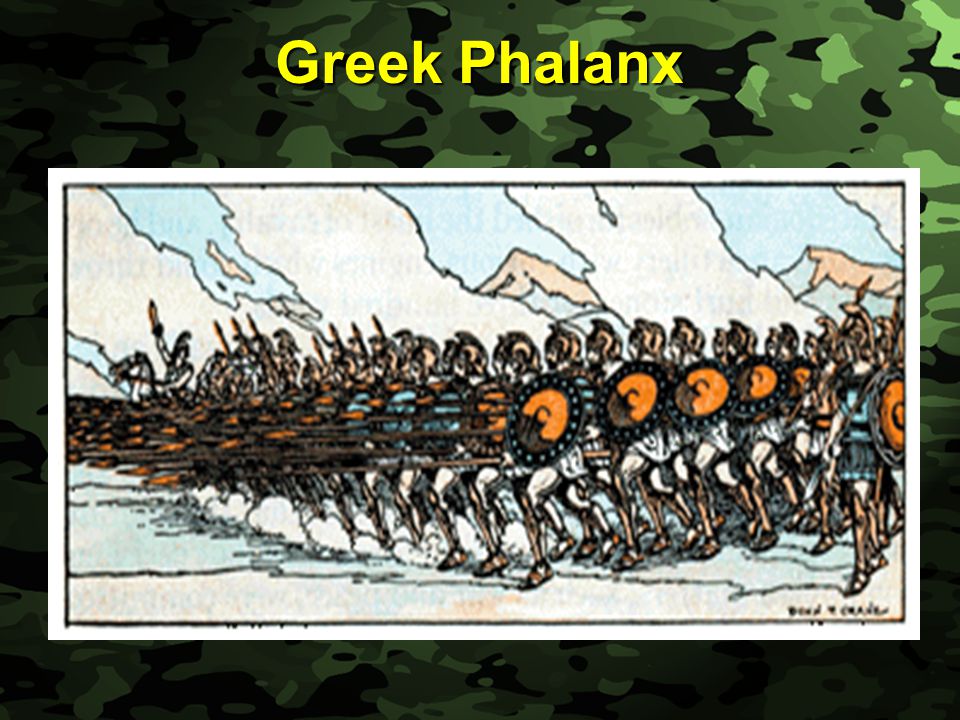The poster artwork features a vibrant camouflage background in various shades of green, dark brown, and black. Bold yellow lettering at the top spells out "Greek Phalanx." The scene depicts troops arranged in regimented rows, facing left, with their spears thrust uniformly in that direction. The spear tips are a striking orange, matching the center of their circular shields, which have blue accents around the edges. Each soldier wears a helmet adorned with a crest resembling a mohawk. Among the infantry, a single soldier rides a white horse, positioned towards the far right of the image. In the middle of the scene, there is a noticeable synergy of orange and blue hues, representative of the soldiers' shields and the surrounding environment, which includes distant mountains and dust clouds rising from beneath their feet. Although obscured, there is text at the bottom of the image hinting at further context beyond the immediate visual elements. The overall impression is one of organized, disciplined warriors in a medieval setting, preparing for battle.